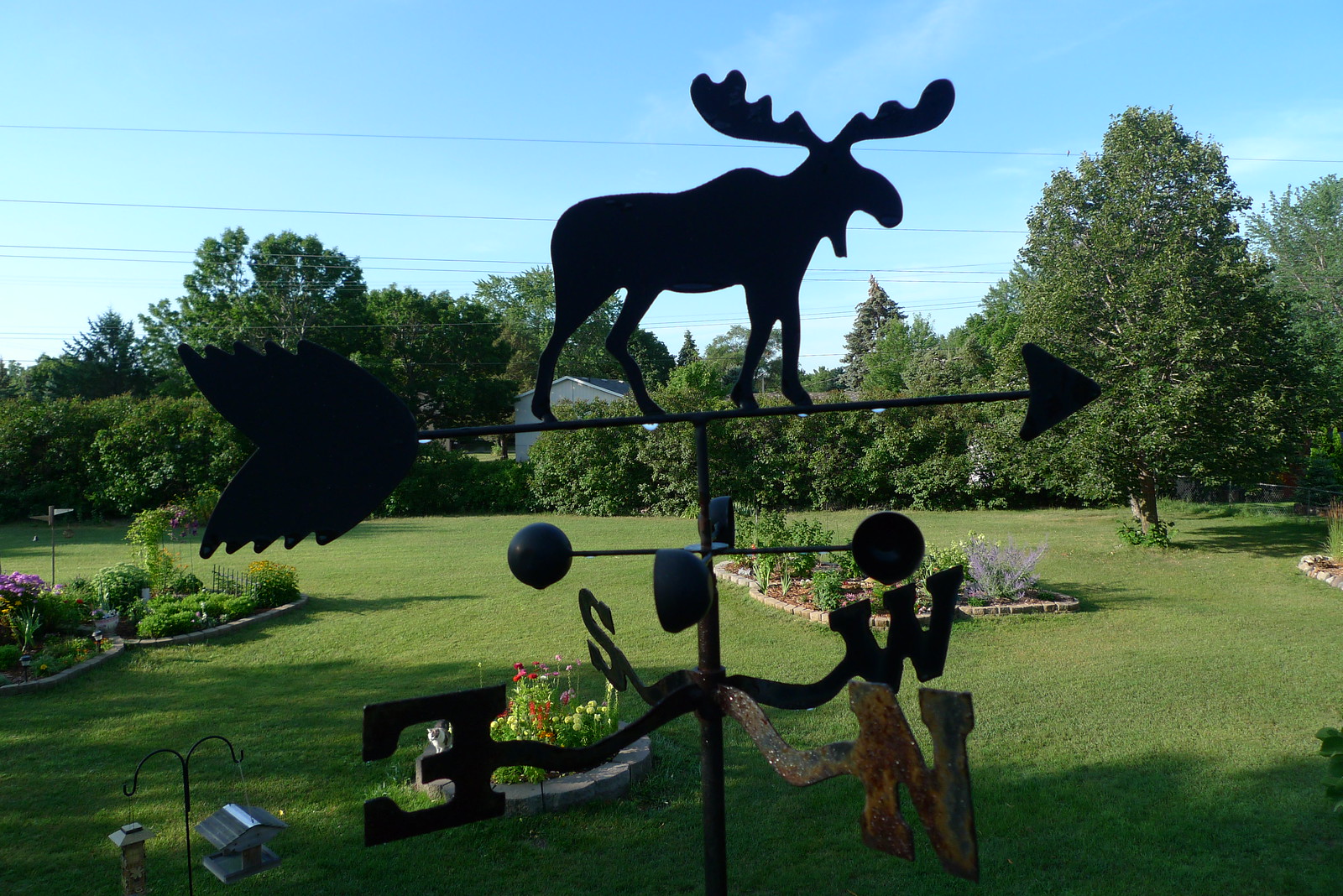This photograph captures a picturesque large garden backyard on a clear day with a blue sky accentuated by wispy white clouds. The focal point of the image is a detailed weather vane situated prominently in the center. The weather vane, crafted from what appears to be black metal, features a silhouetted moose standing atop an arrow. This arrow, designed with a large tail on the left and a pointed tip on the right, is mounted to a vertical rod extending from the ground. Below the arrow, two vertical wires with spherical ends flank four curved metal arms that indicate the cardinal directions—North, East, South, and West—with corresponding letters.

The garden is lush and well-maintained, with a variety of flowers in vibrant hues of purples, blues, pinks, reds, and yellows. These flowers are arranged in distinct garden beds sectioned off by stone pavers. A brown pipe supporting the weather vane emerges from one of these beds, which are spread throughout the yard. To the left, a flower bed features low green shrubs and flowering plants. Towards the back, several stone-paved garden areas offer more floral displays amidst expanses of green grass. A large tree occupies the right-hand corner, while a line of hedges forms the background. Adding to the charm, there are also two birdhouses hanging from shepherd hooks within the garden.